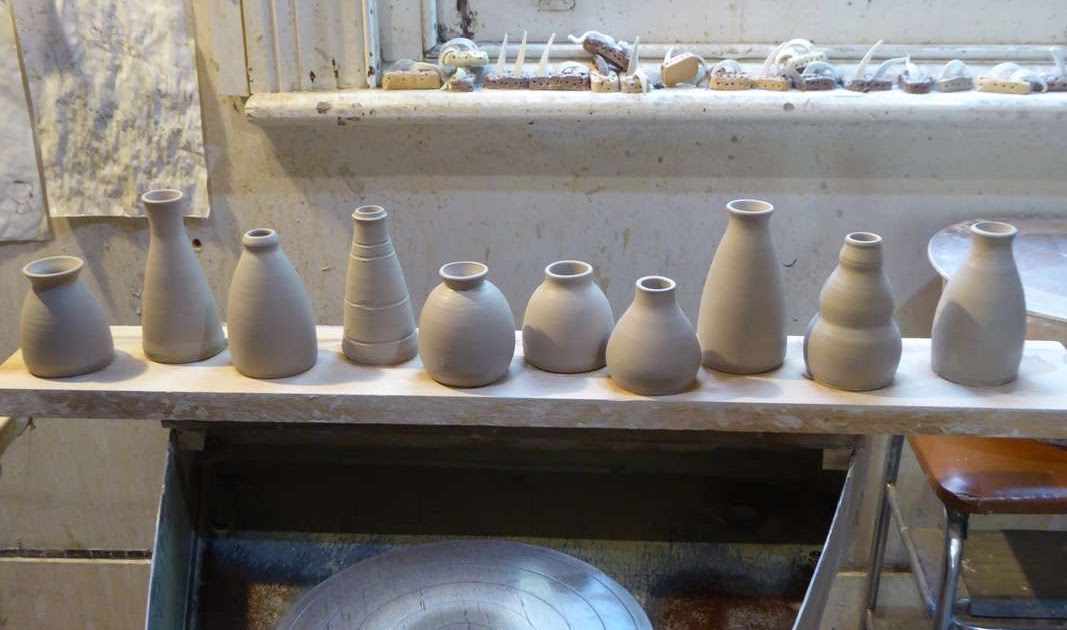In this photograph, taken in what appears to be an art studio, an array of clay pots is meticulously lined up on a wooden board for display. These handcrafted clay vessels, totaling ten, exhibit a variety of shapes and sizes—some are tall and slender, while others are shorter and wider, resembling vases in their form. The background features a white wall, marred with splashes of grayish clay water, hinting at the creative processes that unfold in this space. To the left, one can discern a potter's wheel, a crucial instrument for shaping the clay. Above the wooden board, shelves hold various pottery tools, indicative of the craft evidenced by the pots below. A brown leather-cushioned chair sits in the background, adding a touch of lived-in comfort to this artist's workspace. The overall image exudes a cohesive clay-toned palette, emphasizing the earthy materials central to the scene.